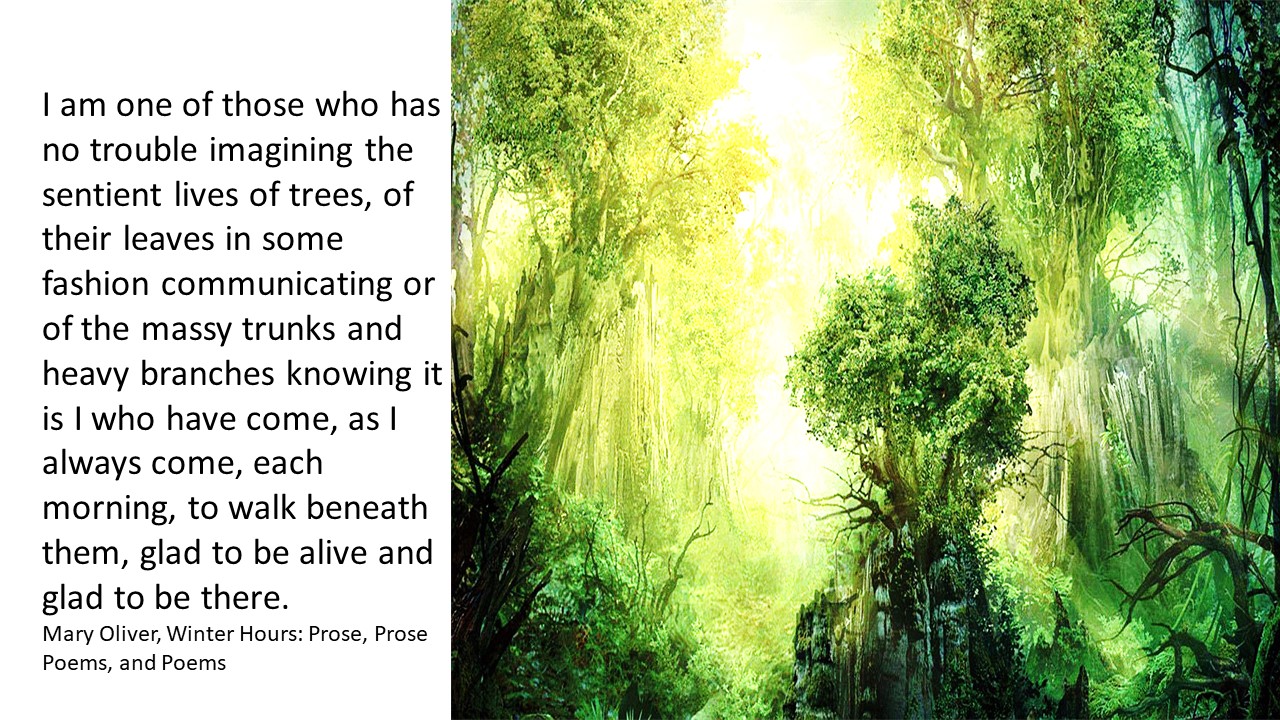The graphic features a surreal depiction of a lush, fantasy forest with unrealistically tall trees and mountains. The branches appear to be almost crawling outwards, creating a fantastical atmosphere illuminated by a bright light in the distance. The forest imagery is heavily saturated with vibrant greens and blues, enhancing its dreamlike quality. On the left side of the image, in black text, is a quote: "I am one of those who has no trouble imagining the sentient lives of trees, of their leaves in some fashion communicating, or of the massy trunks and heavy branches, knowing it is I who have come, as I always come, each morning to walk beneath them, glad to be alive and glad to be there." This quote is attributed to Mary Oliver from her book "Winter Hours: Prose, Prose Poems, and Poems."